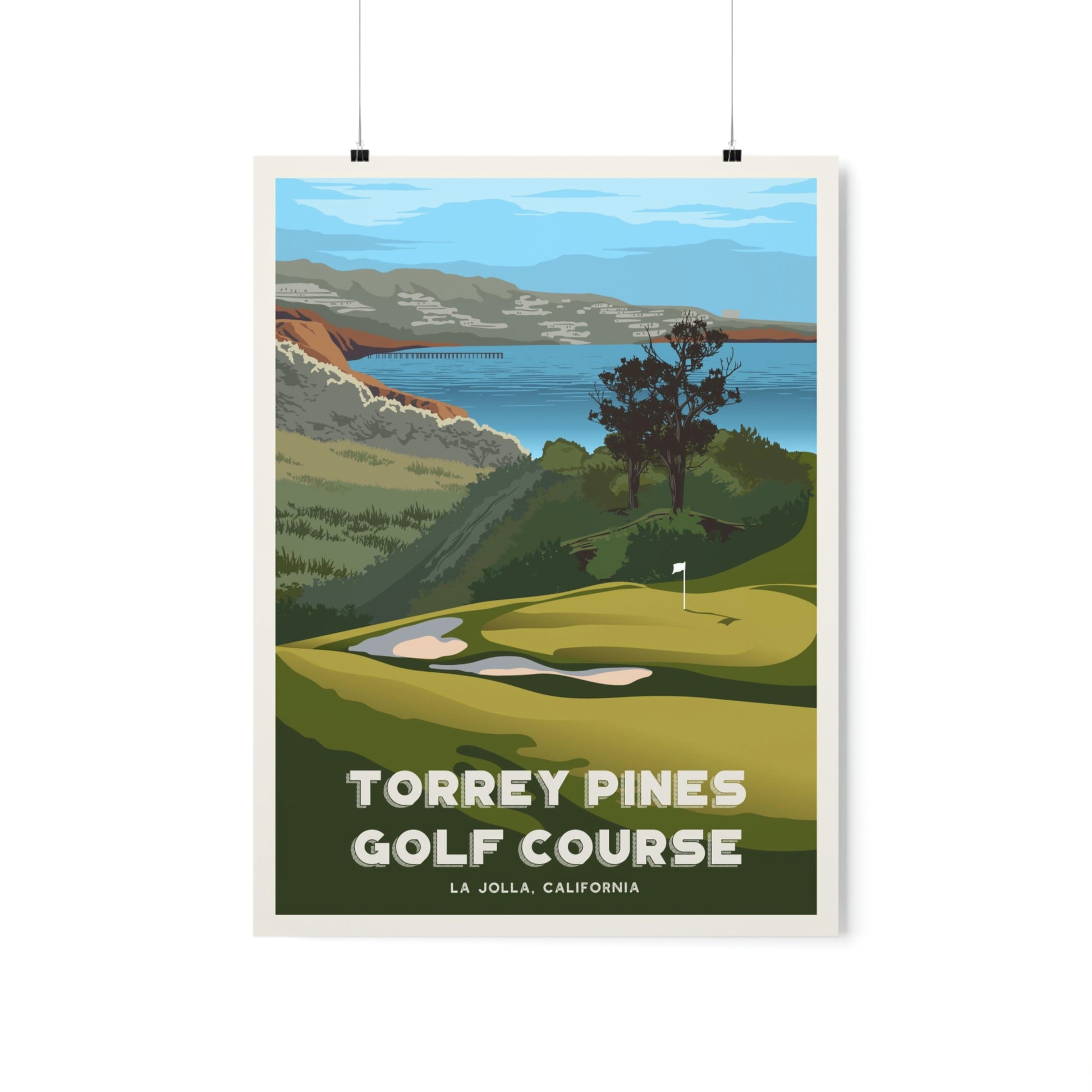This poster, featuring a lush, green-themed digital painting of the renowned Torrey Pines Golf Course in La Jolla, California, captures the serene ambiance of the location with intricate details. The composition centers on a vibrant putting green with a prominent white flag marking the hole, flanked by two white sand bunkers. The landscape extends to showcase rugged mountains adorned with pine trees and a calm, blue water body, likely the ocean or a bay, in the distance. A small black pier juts into the water, adding a quaint touch. Above, layers of clouds in various shades of gray and blue paint a tranquil sky. The poster is framed by a light gray border and is suspended by two black clips connected by a small chain. At the bottom, in crisp white letters, the text reads "Torrey Pines Golf Course," followed by "La Jolla, California" in smaller print, grounding the scene in its real-world locale.